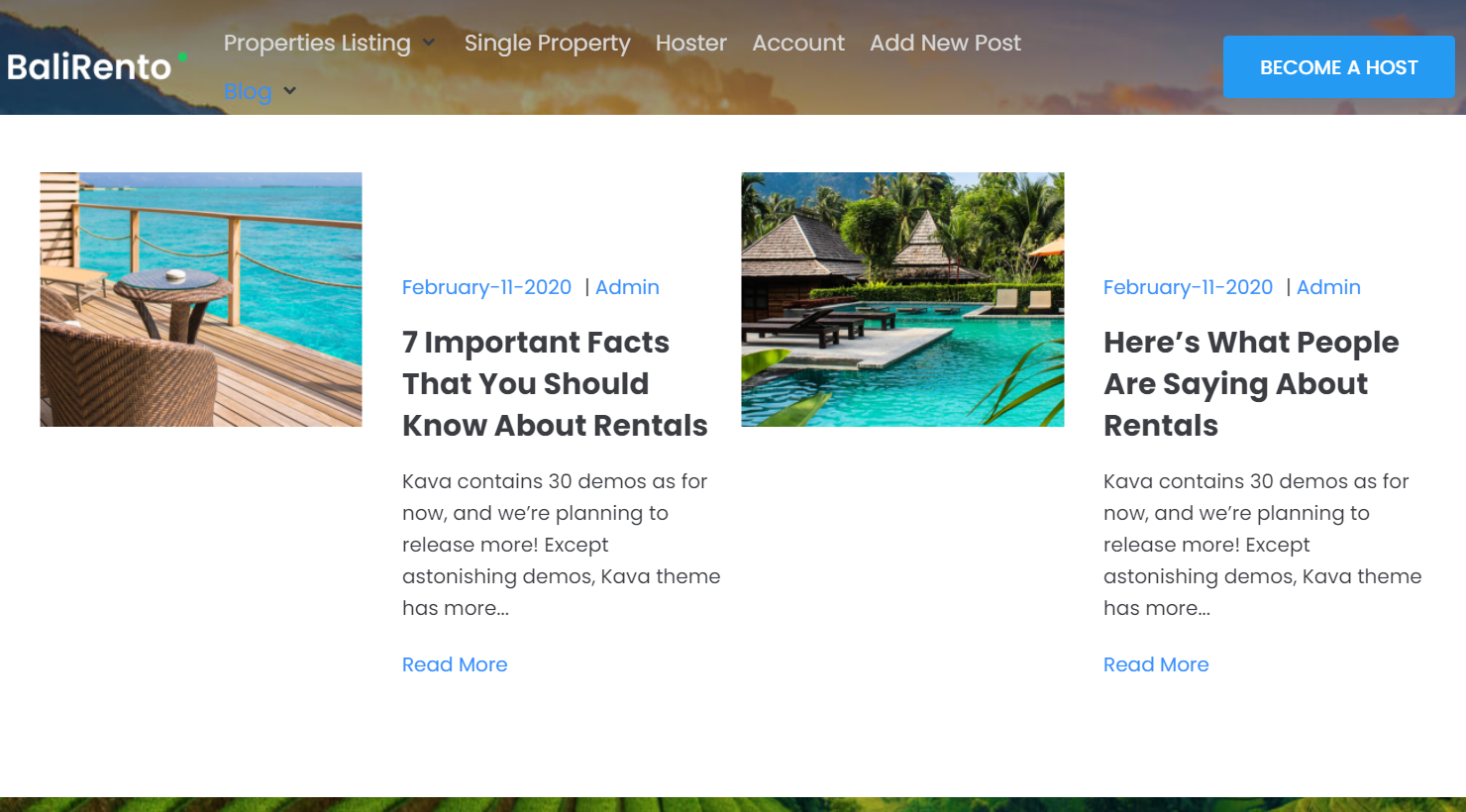This horizontal rectangular image features a top section with a white background displaying the logo "ValleyBALI-RENTO" in capital letters with a small green dot after it. The top also includes a white font menu identifying sections labeled "Properties Listing," "Single Property," "Hoster," "Account," and "Add New Post," all set against a muted backdrop with mountains and clouds to the left.

On the right-hand side, a turquoise rectangular section carries the text "Become a Host" in white font. Moving back to the left, there's a horizontal image depicting a wooden deck with vertical planks. The deck features wrought iron furniture, including a chair and table, and a tan barrier overlooking the ocean. To the right of the image, turquoise or blue font displays "February 11, 2020," followed by "Admin" in black font. Below that, in black font, it reads "Seven important facts that you should know about rentals," with smaller text below stating, "Kava contains 30 demos as for now, and we're planning to release more. Except astonishing demos, Kava theme has more." Just beneath, it says "Read more" in turquoise.

The next column presents another horizontal, rectangular image of a tropical setting featuring thatched huts, varied seating arrangements around a beautiful blue-green pool, and tropical trees in the background. Adjacent to this image, blue text again reads "February 11, 2020," followed by "Admin" in black font. Below, in black font, it states, "Here's what people are saying about rentals. Kava contains 30 demos as for now, and we're planning to release more. Except astonishing demos, Kava theme has more," with a turquoise "Read more" beneath.

At the very bottom, a thin rectangular stripe spans from left to right, featuring green hues likely derived from the plant-filled images above.